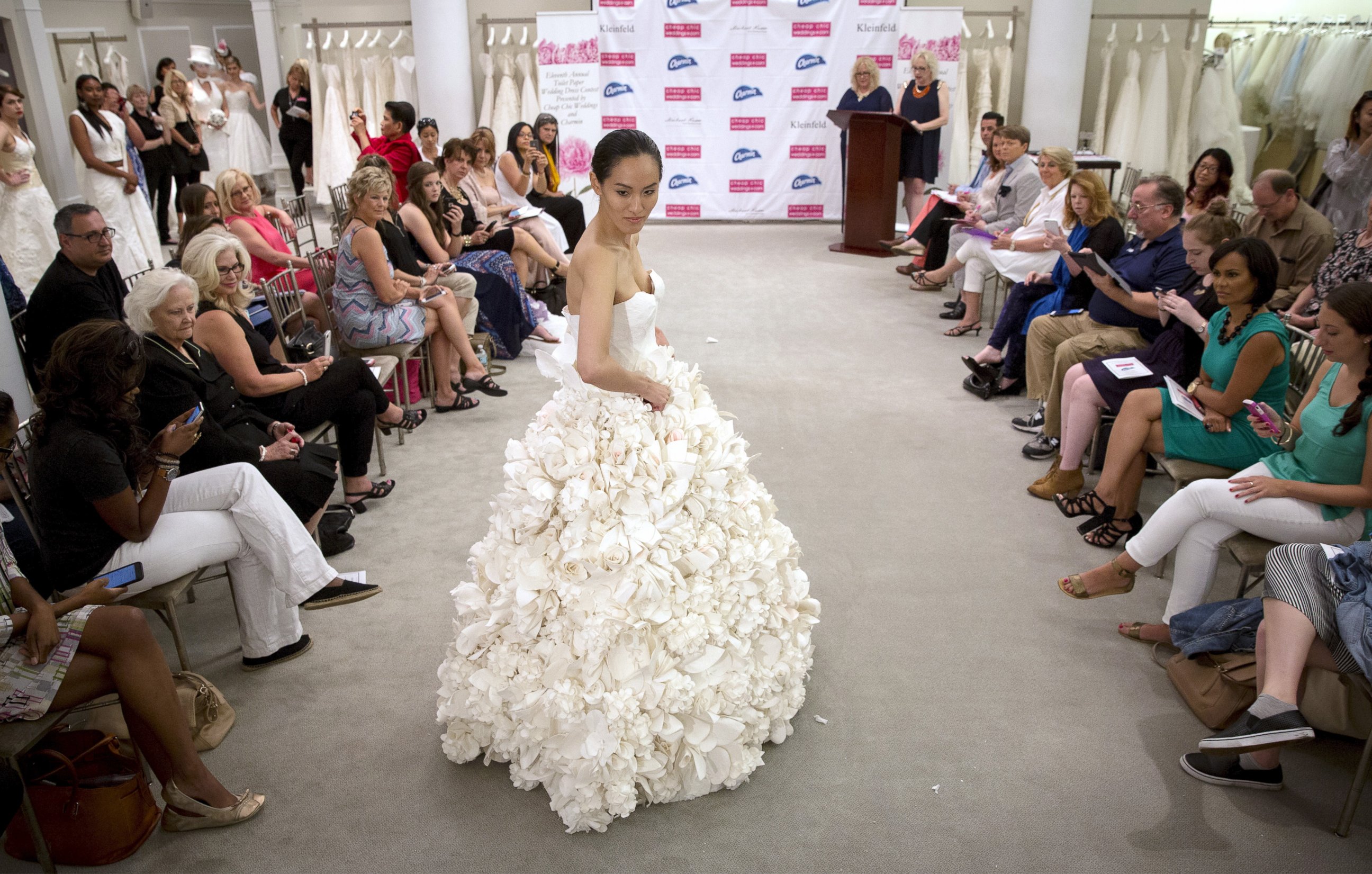The photograph captures a runway show centered around wedding dresses. The focal point is a model in a stunning white, strapless wedding gown characterized by a fitted bodice that flares into a voluminous, flower-like skirt made of intricately gathered fabric resembling roses. The model, with dark brown hair styled up, stands toward the end of the gray runway, looking over her shoulder as she starts to turn around. Audience members, dressed in elegant attire, line both sides of the runway, seated in gilded, wooden chairs, some taking notes and others holding invitations or programs on their laps. In the background, more models, dressed mostly in white wedding gowns, are awaiting their turn. A white banner adorned with red and blue boxes and unreadable text hangs at the rear, while two officials, a man and a woman, stand behind a wooden podium, likely announcing the dresses. The setting is bustling, with additional wedding dresses hanging on racks, contributing to the event's vibrant and festive atmosphere.